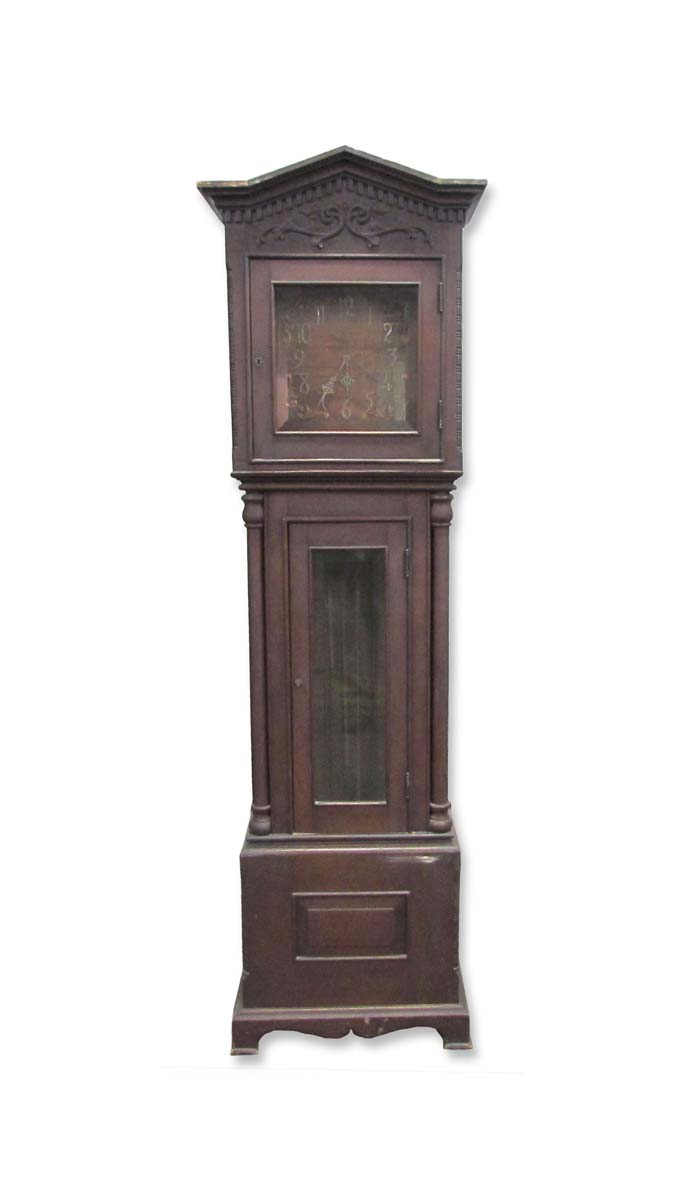A detailed photograph showcases an antique grandfather clock, set against a plain white background, devoid of any visible borders. This tall, rectangular-shaped clock stands approximately five feet tall and one and a half feet wide, with a wooden construction featuring intricate craftsmanship. The clock’s face, framed by a glass door, displays Arabic numbers in a dark golden-bronze hue, set against a dark brown wooden backdrop. Above the clock face, the top portion of the structure mimics a gable-like roof with slightly elevated wings, adorned with elaborate bas-relief filigree and floral carvings. The middle section of the clock, the tallest part, features a cabinet-like enclosure with a glass door revealing what appear to be metal rods, possibly part of the clock’s chime mechanism. Below this, a lower square door allows access to components for winding the clock. The clock rests on four sturdy feet, completing its elegant, timeworn presence.